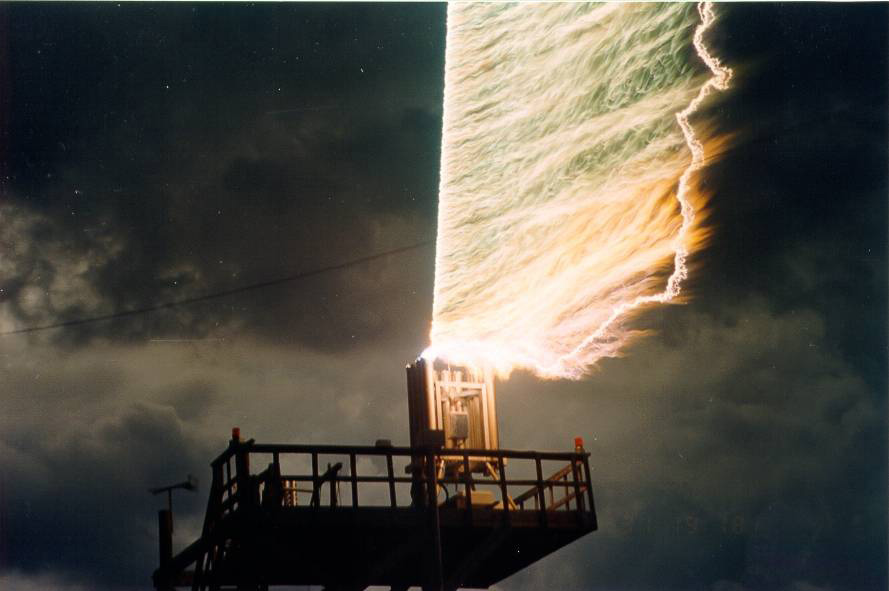A nighttime scene captures the dramatic moment a powerful lightning strike hits an elevated platform, presumably equipped with an electrical box or lightning rod. The intense electrical discharge, descending from the stormy, cloud-filled sky, appears to have struck with force, illuminating the surrounding darkness with a vivid, fiery explosion. Electromagnetic plasma, predominantly glowing in shades of orange with tinges of green, radiates from the impact point, creating a mesmerizing display that snakes around the boundaries of the platform. The spectacle of light and energy is both striking and chaotic, hinting at the raw power of nature, whether this phenomenon was by accident or design remains a mystery.